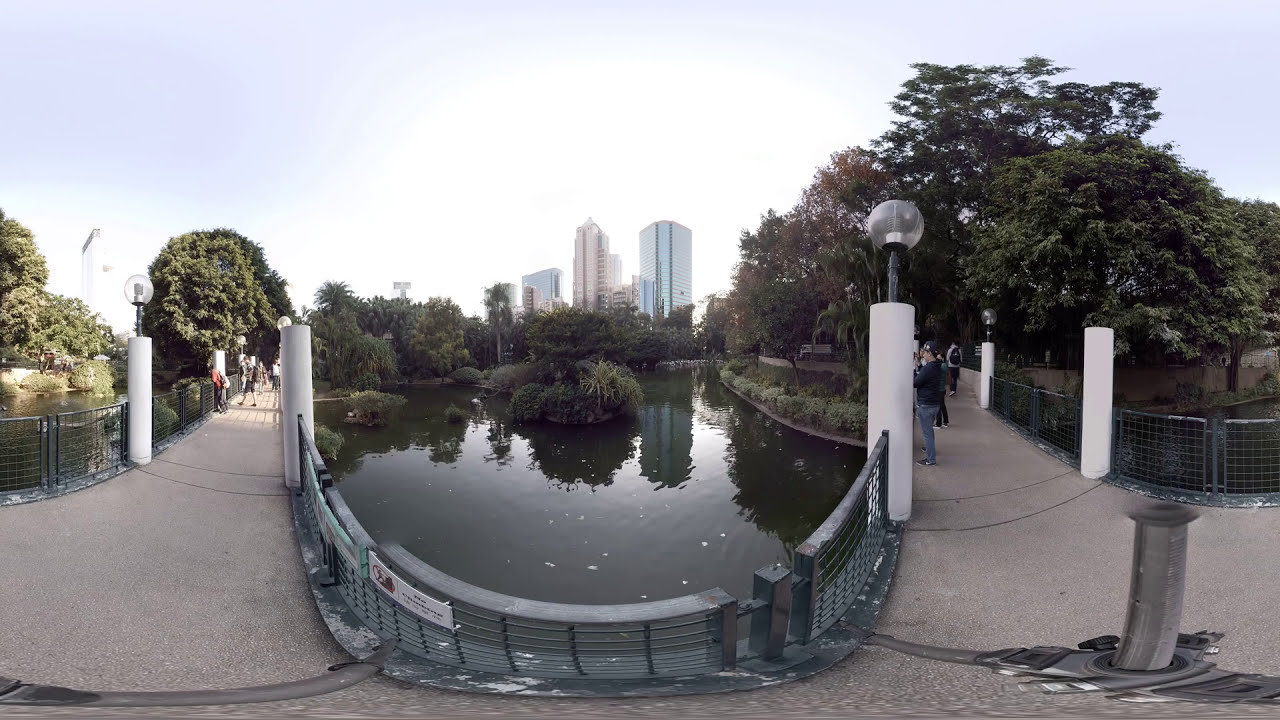In this detailed photo, we see a serene pond nestled in the middle of a large city park, bordered by walkways on both its left and right sides. The pond is graced with small islands adorned with bushes and plants, and even a tree growing out from one of these islands. The walkways, which seem to wrap around the pond in a U-shape, are fenced off from the water, with light poles lining the paths. These light poles have a white base, a black middle, and a silver glass sphere on top. On both sides of the pond, several people are seen strolling or observing the picturesque scene, including one gentleman who appears to be taking a photo of the pond. The park is lush with trees, including a large shade tree on the right side that stretches over the walkway. In the distance, city buildings rise against a cloudy yet sunny sky, creating a striking backdrop. A pipe is visible at the very forefront of the image. Overall, the picture captures a peaceful, green oasis amid an urban setting.